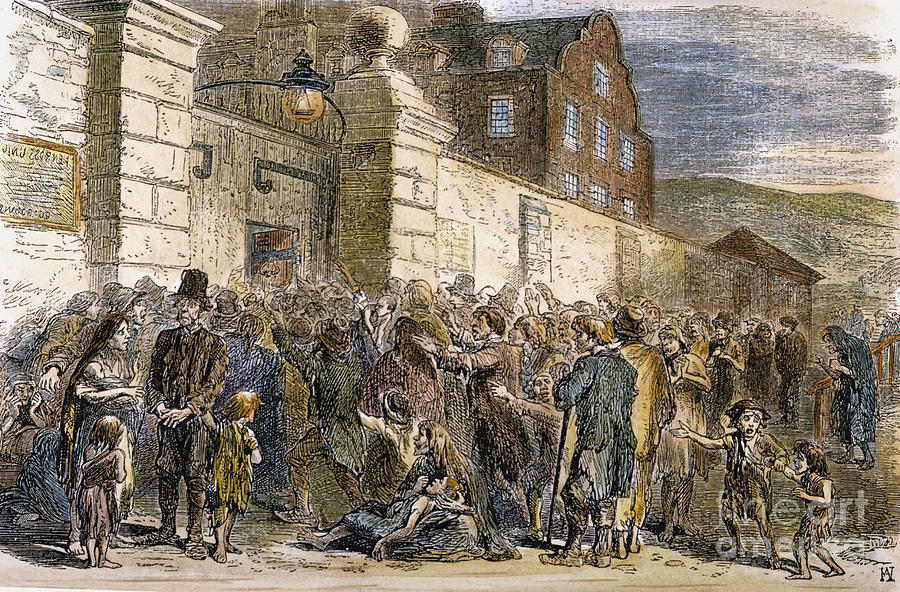This detailed and vibrant illustration, reminiscent of 19th-century book art, portrays a poignant scene from the 1840s, likely during the Great Potato Famine. The top half of the image is dominated by an elaborate stone wall with ornate pillars framing an impressively tall and sturdy wooden gate, adorned with oversized cast iron hinges. A wrought-iron lantern is suspended above the gates, adding a touch of elegance. Attached to the right-hand door is a paper notice, contrasting with the brass plaque on the left pillar, likely providing information about the building. 

In front of this formidable entrance, a large and distressed crowd, representing a cross-section of society, including gentlemen in top hats and black morning coats, children, and visibly frail figures, jostles to gain entry. The crowd's expressions range from anger to desperation, unified in their urgent need to pass through the gate. Notably, a woman clutching a baby and another seated with her child stand out in the foreground, highlighting the widespread suffering.

The artwork captures the tension and despair of the crowd, with many arms raised in supplication or protest. The sense of urgency is palpable, although slightly blurred by the artistic style. In the bottom right corner, a faint watermark reads "Fine Art," hinting at the piece's quality and age.